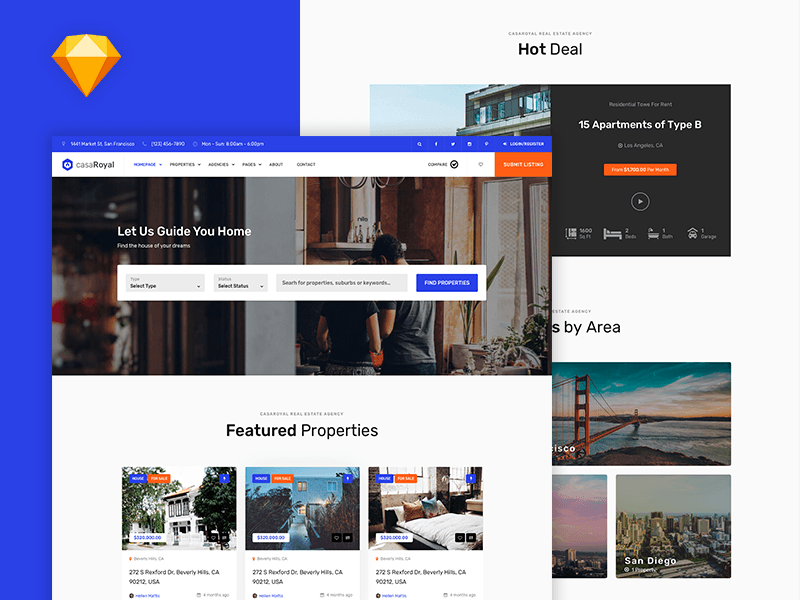**Detailed Image Caption:**

The screenshot depicts a tablet displaying an interface of a property search website or application with a contemporary and user-friendly design. The background is primarily white, featuring various photos of properties arranged in an aesthetically pleasing manner within overlaid blocks that offer detailed information when interacted with.

A significant vertical section on the left, approximately one-third to two-thirds of the page, is highlighted in medium blue and prominently displays a gold diamond icon or logo at the upper left corner. This section overlays part of the background and adds visual interest to the layout.

Dominating the central portion of the screen is a pop-up section styled as a distinct page, complete with its own top menu. The section features a blue border on top followed by a white border, housing the blueprints and the brand name "Casa Royal." The menu includes links such as New, Page, Properties, Address, Prices, About, and Contact. Below the menu, against an inviting indoor photo of a cozy apartment room, is a white text caption asserting "Let us guide you home." This caption is accompanied by a property search text box and a blue "Find Properties" button. Beneath this main section, there are thumbnails for three featured properties set against a white background.

To the right of this central overlay, partially obscured by it, the page continues with additional content. The heading "Hot Deal" is prominently placed towards the upper middle right, followed by a black section highlighting "15 apartments of type B" along with a truncated image of an apartment. Below this, a segment labeled "By Area" features small truncated thumbnails of locations, including recognizable cities like San Francisco, with a glimpse of the Golden Gate Bridge, and San Diego. A small, partially covered thumbnail appears adjacent to the featured properties section, though its details are obscured.

Overall, the interface is visually rich and thoughtfully organized, offering users an engaging browsing experience for property searching.